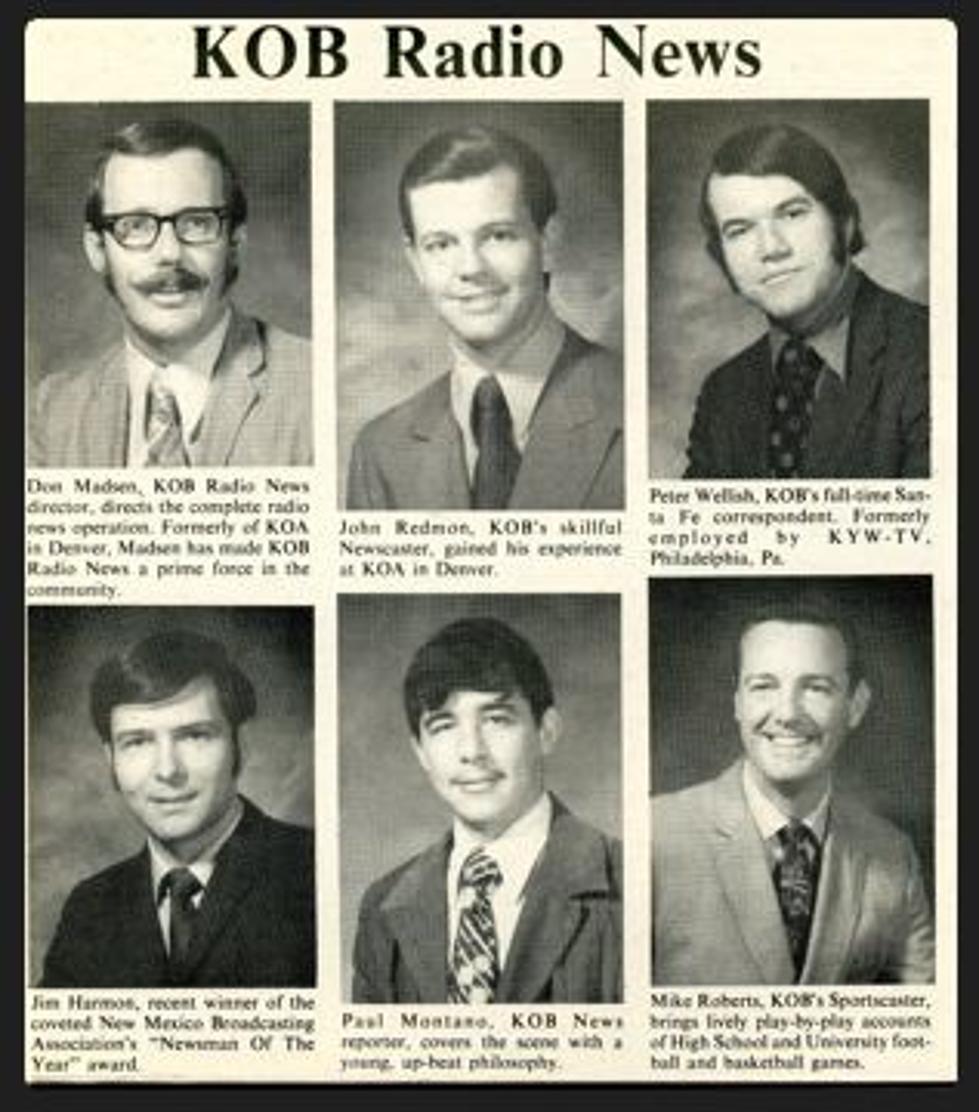The image is a sepia-toned portrait of six male newscasters from KOB Radio News, arranged in two rows of three against a white background with a black border. Each man is captured from the top of his head to the middle of his chest, all donning professional suits and ties. The top row features Don Madsen, the director with dark hair, black glasses, and a moustache; John Redmond, a newscaster with brown hair; and Peter Wellish, the correspondent. The bottom row includes Jim Harmon, another newscaster; Paul Montano, a reporter; and Mike Roberts, the sportscaster. Each portrait is accompanied by a brief description of their role and background in a black serif-style font, enhancing the professional and vintage aesthetic of the radio news team's presentation.